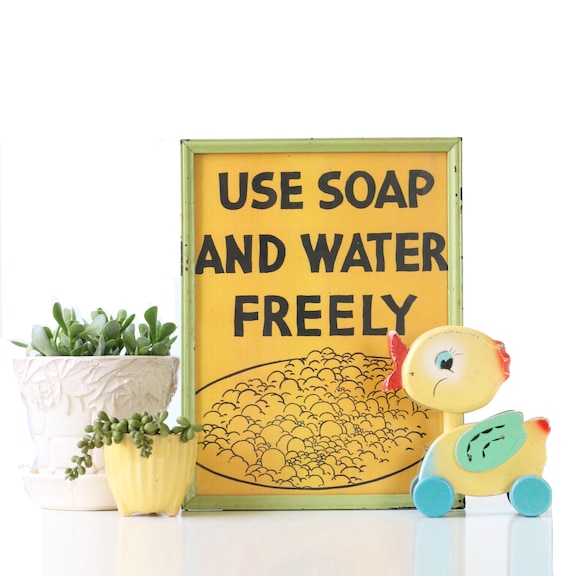The image displays a bright and clear scene on a shiny white countertop, where four objects are arranged in a stylized manner. On the left side, there are two green succulent plants: a larger one in a white pot and a smaller one in a yellow ceramic cup, positioned closer to the center. At the center of the image stands a framed sign with a light green frame and an orange background. The sign prominently features the black, all-capitalized text "USE SOAP AND WATER FREELY" above an illustration of a bubbling sink. To the right, there is a vintage wooden duck toy on wheels. The duck is vividly colored in yellow, light blue, green, and red, with details such as a blue eye, red beak, and red accents on its head and tail. The entire arrangement reflects clearly on the glossy countertop, enhancing the overall brightness and clarity of the setting.